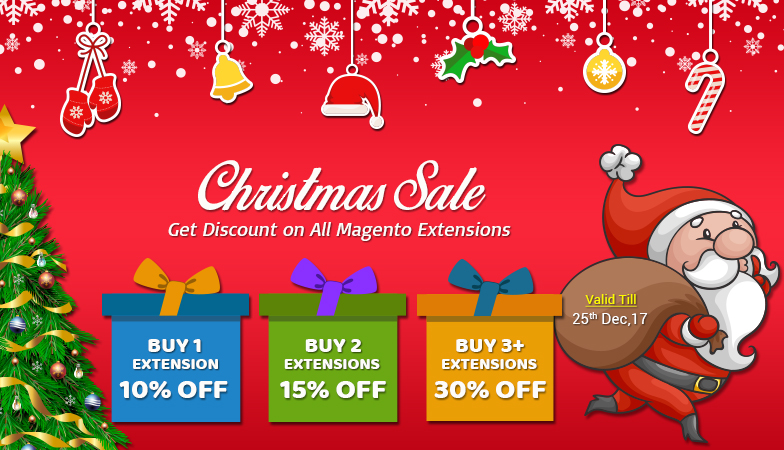The homepage of the Christmas sale website is adorned with festive elements and vibrant colors, highlighting the special discounts on all Magento extensions. 

At the top of the page, there is a flurry of white snowflakes gracefully falling against a striking red background, setting a cheerful holiday mood. Complementing this, white strings dangle a variety of Christmas decorations, including red mittens, a golden bell, a Santa's hat in classic red and white, a sprig of holly in green and red, a delicate ornament, and a candy cane.

Towards the bottom of the screen, three gift boxes in vivid shades of blue, green, and yellow offer enticing discounts: 
- The blue box announces "Buy one extension, get 10% off."
- The green box proclaims "Buy two extensions, get 15% off."
- The yellow box boasts "Buy three or more extensions, get 30% off."

A jolly Santa Claus in the right-hand corner adds to the festive spirit. He is depicted in traditional attire with black boots, a black belt, a red hat, a white beard, mustache, and eyebrows. Over his shoulder, he carries a brown sack that reads, "Valid till the 25th of December 2017."

In the left-hand corner stands a beautifully decorated Christmas tree, adorned with a gold star at the top and elegant gold ribbons, epitomizing the joyous holiday season.